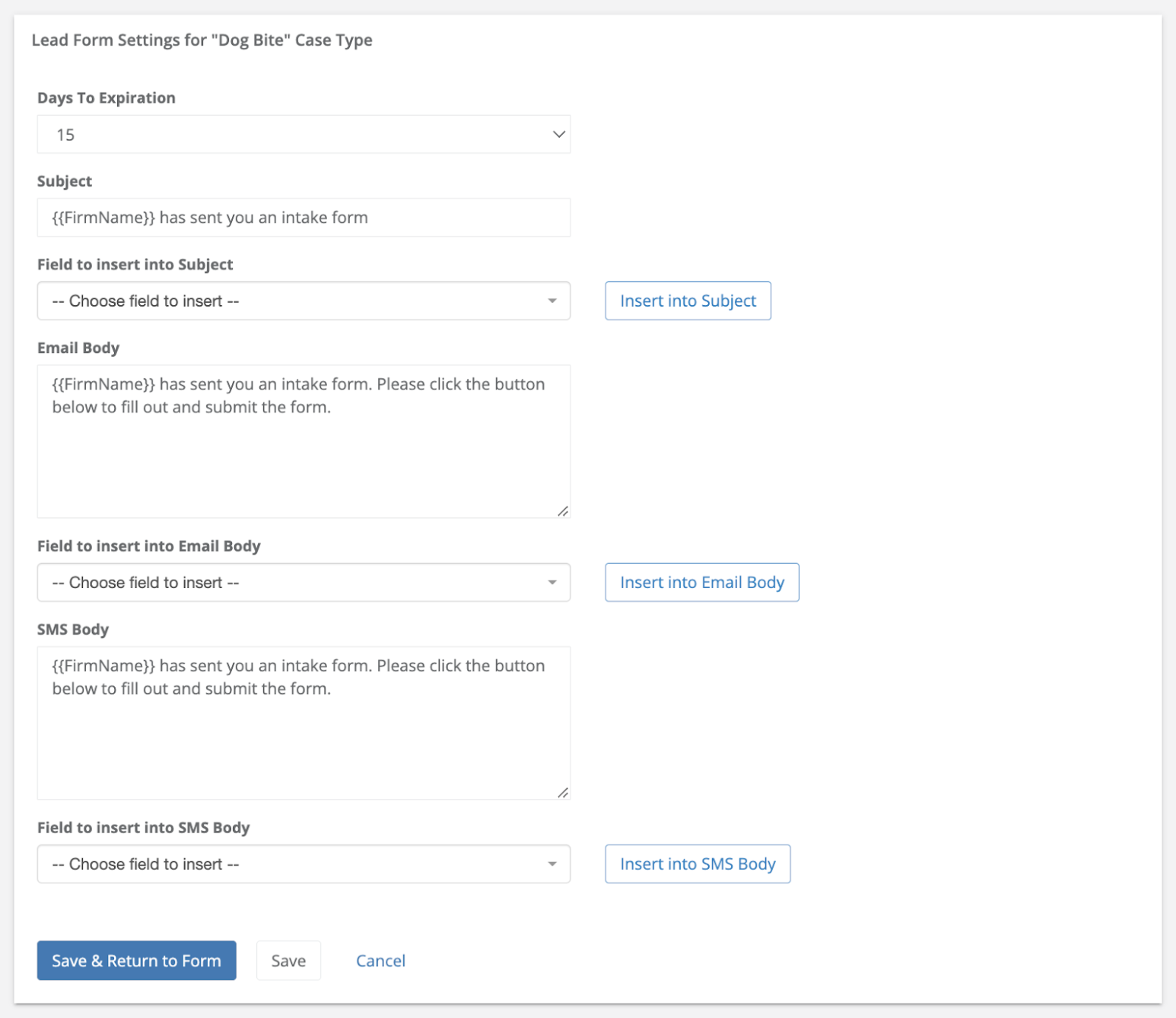The image depicts a website hosting a fillable form designed to report incidents. This pro forma document is used to collect detailed information about incidents, though its exact recipient, such as law enforcement or personal documentation, is not clearly indicated. 

At the top left corner of the form, there is a small black font label that reads "Lead Form Settings for 'Dog Bite' Case Type." Following this, there is a field labeled 'Days to Expiration,' indicating the user has a limited timeframe to complete the form. The next component is the 'Subject Line,' which requires the user's first name or firm name. 

Beneath the subject line is a field titled 'Insert into Subject,' equipped with a drop-down menu offering various subject options. The form also includes a section labeled 'Email Body,' where users can describe the details of the incident comprehensively. Additional drop-down menus are available to include further relevant information or specifics pertaining to the incident report.